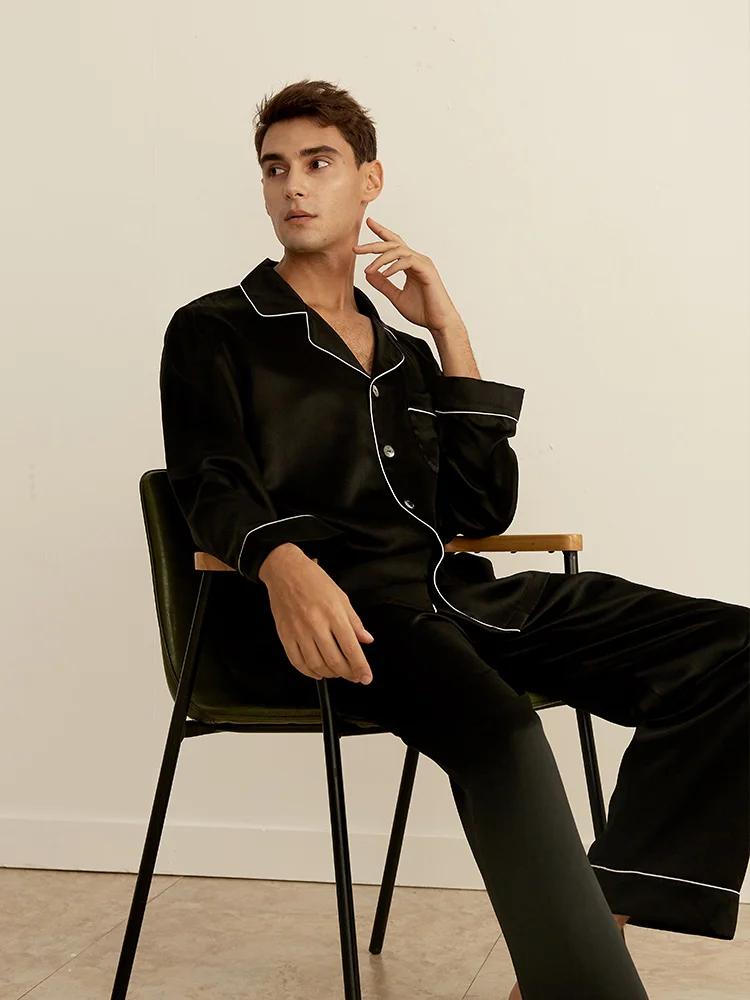This rectangular photograph, taken indoors, depicts a young man in his 20s seated in a modest, black-frame chair with a green back and seat cushion, detailed with tan wooden armrests. The man, with short brown hair combed back and brown eyes, sits with his body angled towards the right side of the image, while his head is turned left, giving a contemplative air. Dressed in luxurious black velvet pajamas accented with white piping along the collar, button-up front, and cuffs, he rests his right arm comfortably on the armrest. His left arm is raised near his face, with his elbow resting on the chair's armrest. The flooring beneath him features large square tiles in tan and gray hues, lending a sophisticated yet casual ambiance to the room. An eggshell or cream-colored wall forms the backdrop, completing the relaxed and understated setting of the photograph.